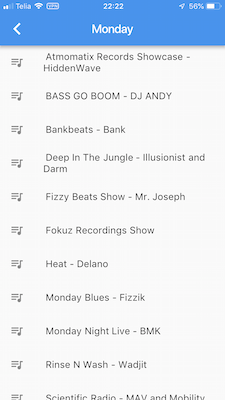This image is a screenshot taken from a mobile phone displaying a list of music tracks. The screenshot was taken at 10:22 PM, as indicated in the status bar at the top. The phone is connected to the Telia network and has a 56% battery charge remaining. Notably, location services are enabled. 

At the very top, there's a blue banner with white text that reads "Monday," including a back arrow icon also in white. Below this banner, a list of music tracks is displayed. Each song entry is accompanied by an icon on the left side, featuring a music note beside three horizontal lines, likely indicating that the tracks can be rearranged in a playlist.

The listed tracks include:
1. **AUTOMATIX RECORDS SHOWCASE - HIDDEN WAVE**
2. **BASS GO BOOM - DJ ANDY**
3. **BANK BEATS - BANK**
4. **DEEP IN THE JUNGLE - ILLUSIONIST & DARM**
5. **FIZZY BEATS SHOW - MR. JOSEPH FOKUS RECORDINGS SHOW**
6. **HEAT - DELANO**
7. **MONKEY BLUES - PHYSICS**
8. **MONDAY NIGHT LIVE - BMK**
9. **RINSE AND WASH - WADJET**
10. **SCIENTIFIC RADIO - MAV & MOBILITY** (partially cut off)

The background of the list is white, with the text rendered in black.